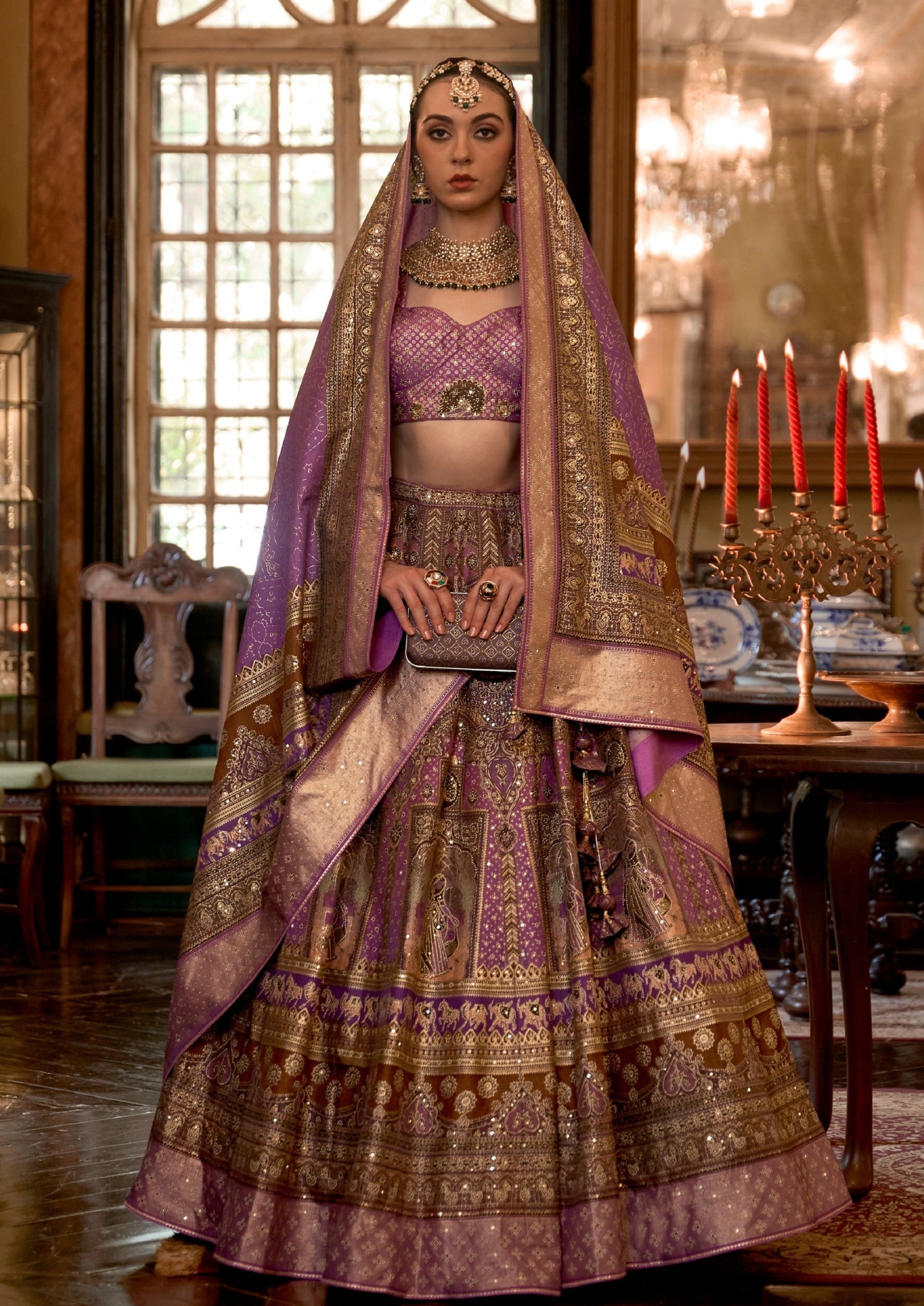In the detailed and highly ornate image, a young woman with brown skin and expressive, large brown eyes is depicted standing gracefully. She wears a flowing, traditional Indian ensemble, characterized by its rich hues of purple, brown, and gold. The outfit features a striking bra-like top adorned in a mix of purple and white, ending just above her midriff. A thick, gold necklace drapes elegantly from the base of her neck down to her chest, revealing a glimpse of skin between her chest and breasts. Complementing her attire is a voluminous, floor-length dress that cascades in circular stripes and rectangular patterns from just above her belly button to her feet. 

Her head is adorned with a long, flowing headscarf that extends from her head down to her waist, partly covering her shoulders and arms. A decorative emblem sits prominently on her forehead, adding to the intricate details of her attire. She stands with her hands clasped in front of her, holding a gray-colored pocketbook, and her fingers, adorned with large rings, point downward.

The backdrop features a setting with a hardwood floor, a large window with a grid pattern on the left, a wooden chair, and a stand holding five orange-lit candles on the right. The environment, combined with the woman's elegant attire and serene, expressionless gaze, suggests a scene from a graphical rendering, possibly from a computer game, evoking a sense of lifelike traditional charm.